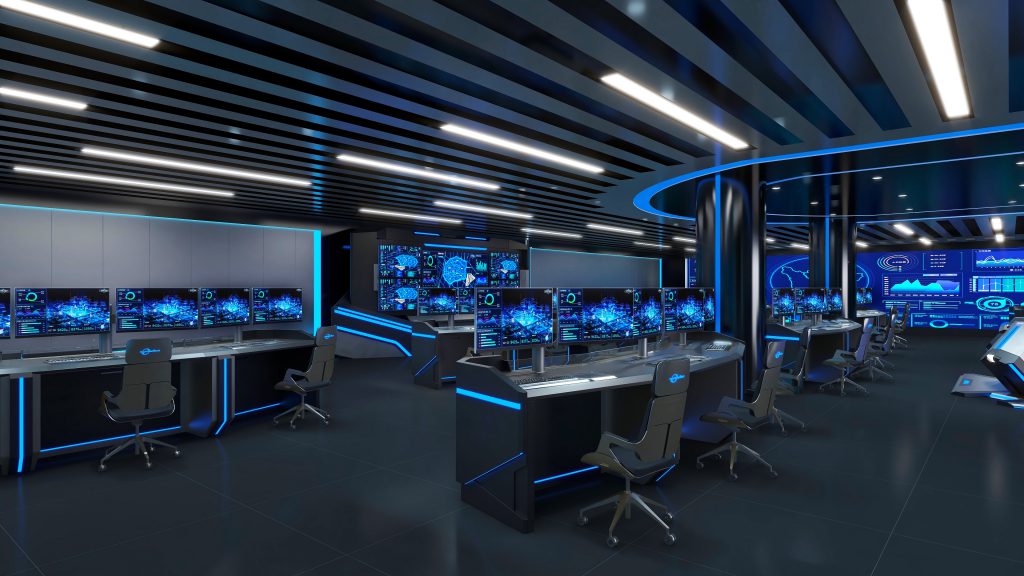The image depicts a high-tech computer lab brimming with desks, computers, and chairs, all arranged in a modern, futuristic setting. The room is characterized by a pervasive blue theme, featuring screens displaying various shades of blue, from light to dark, often filled with intricate line graphs or data visualizations. Blue lights accentuate the desks, chairs, and walls, complementing the contemporary aesthetic. The ceiling is adorned with gray and blue stripes, interspersed with white lights that contribute to the sleek ambiance. Notable architectural elements include silver, futuristic support columns and large black floor tiles. A prominent feature is a massive screen at the back of the room, likely used for data display or presentations, reinforcing the high-tech vibe. The chairs, with high backs and illuminated logos, along with the orderly rows of desks and monitors, all face towards this central screen, suggesting a focus on data analysis or presentations. The overall design gives an impression straight out of a cutting-edge sci-fi movie, blending varying shades of blue, black, and gray to create a sophisticated, high-tech environment.